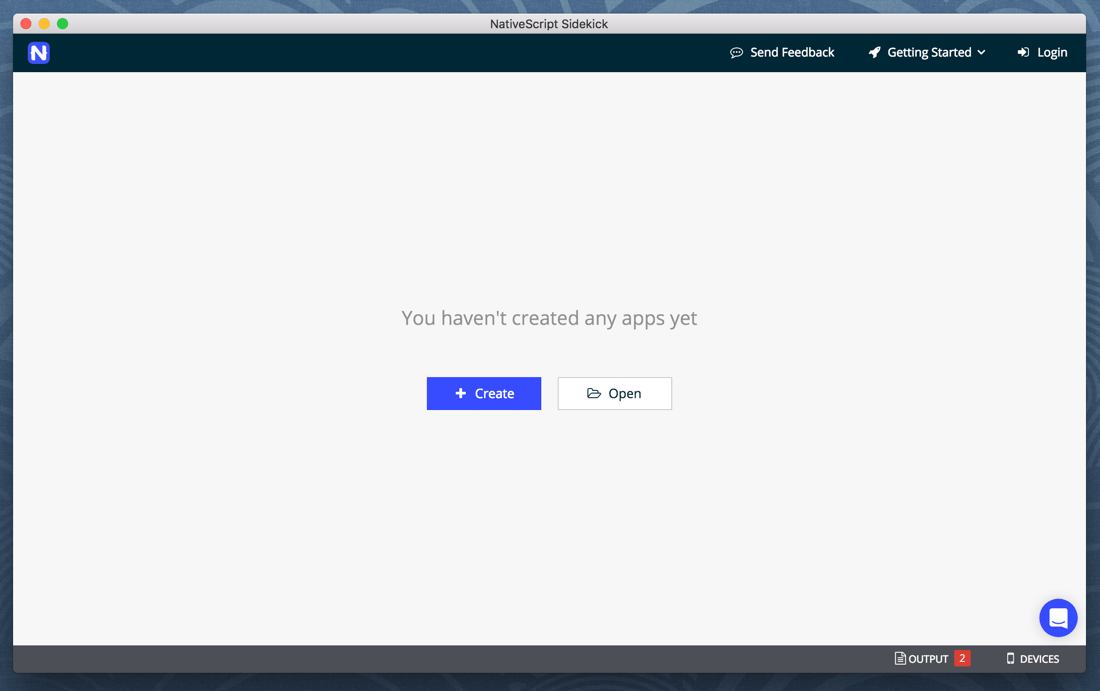The image displays the Native Script Sidekick application interface. At the very top, there is a long text bar with the title "Native Script Sidekick," with the "N" and "S" being capitalized. To the left, there are three colored circles: red, yellow, and green. Below, there's a large blue circle featuring the letter "N." 

Towards the right, there are options for user actions. First, a speech bubble with three dots inside, labeled as "Send Feedback." Next to it is "Getting Started," followed by "Log In" with an arrow pointing to the right.

In the center of the screen, light gray text reads, "You haven't created any apps yet." Beneath this message, there's a prominent blue rectangle with the word "Create" accompanied by a plus symbol. Another option beside it says "Open."

On the far right, there's a small blue circle with an image resembling a piece of white notebook paper inside. Underneath this, the option labeled "Output" appears, next to a red square with the number two inside. Finally, to the right, there's an icon of a cell phone next to the uppercase word "DEVICES."